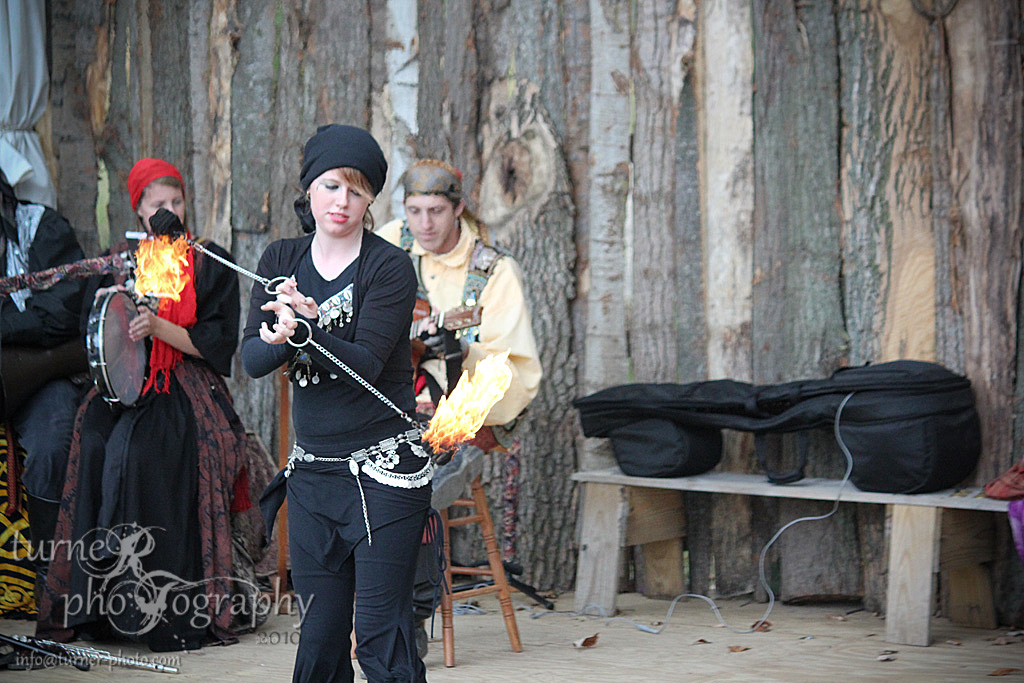This 2010 photograph by Turner Photography captures a lively scene of performers in a rustic, wooded setting, featuring a background of freshly cut wooden walls. The image includes a woman near the center, possibly a teenager, dressed in black pants and adorned with belly-dancing type jewelry on her top and waist. She wears a black headscarf and is shown expertly juggling fire with chains. To her left, another performer, a woman with a red headscarf, plays a drum. There's a half-visible man at the left edge and a man in cultural attire playing a guitar in the background. The overall theme suggests a blend of gypsy and pirate elements, creating an old-time performance atmosphere. A bench and a bag, likely for instruments or performance tools, sit to the right. The watermark confirms the photographer as Turner Photography, with the email information at turnerphoto.com.